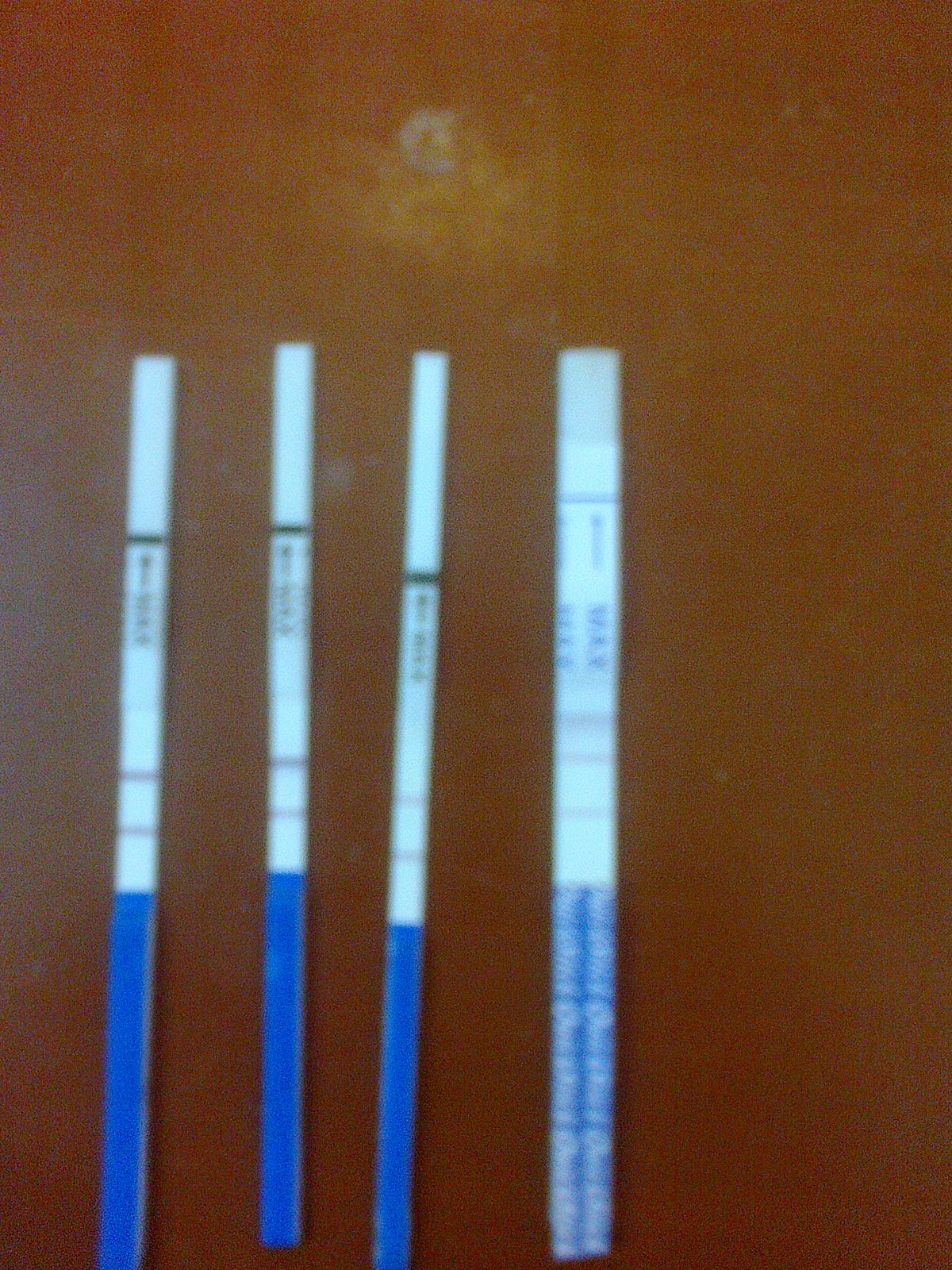The image, though blurry, depicts four paper test strips aligned horizontally, presumably for some form of diagnostic testing. The three test strips on the left are uniformly designed and display identical results. Each of these strips features a white top section with an arrow indicating the proper orientation. Below the arrow, two distinct red lines are present, followed by a solid blue color occupying roughly the bottom third of the strip. 

The fourth test strip on the right is noticeably thicker and similarly has a white top with an orientation arrow. This strip, however, diverges by possibly showing three red lines instead of two; though the blur makes it difficult to ascertain with certainty, there are definitely at least two red lines visible. The bottom third of this thicker strip is also solid blue, but it includes some form of writing that is indiscernible due to the image's lack of clarity.